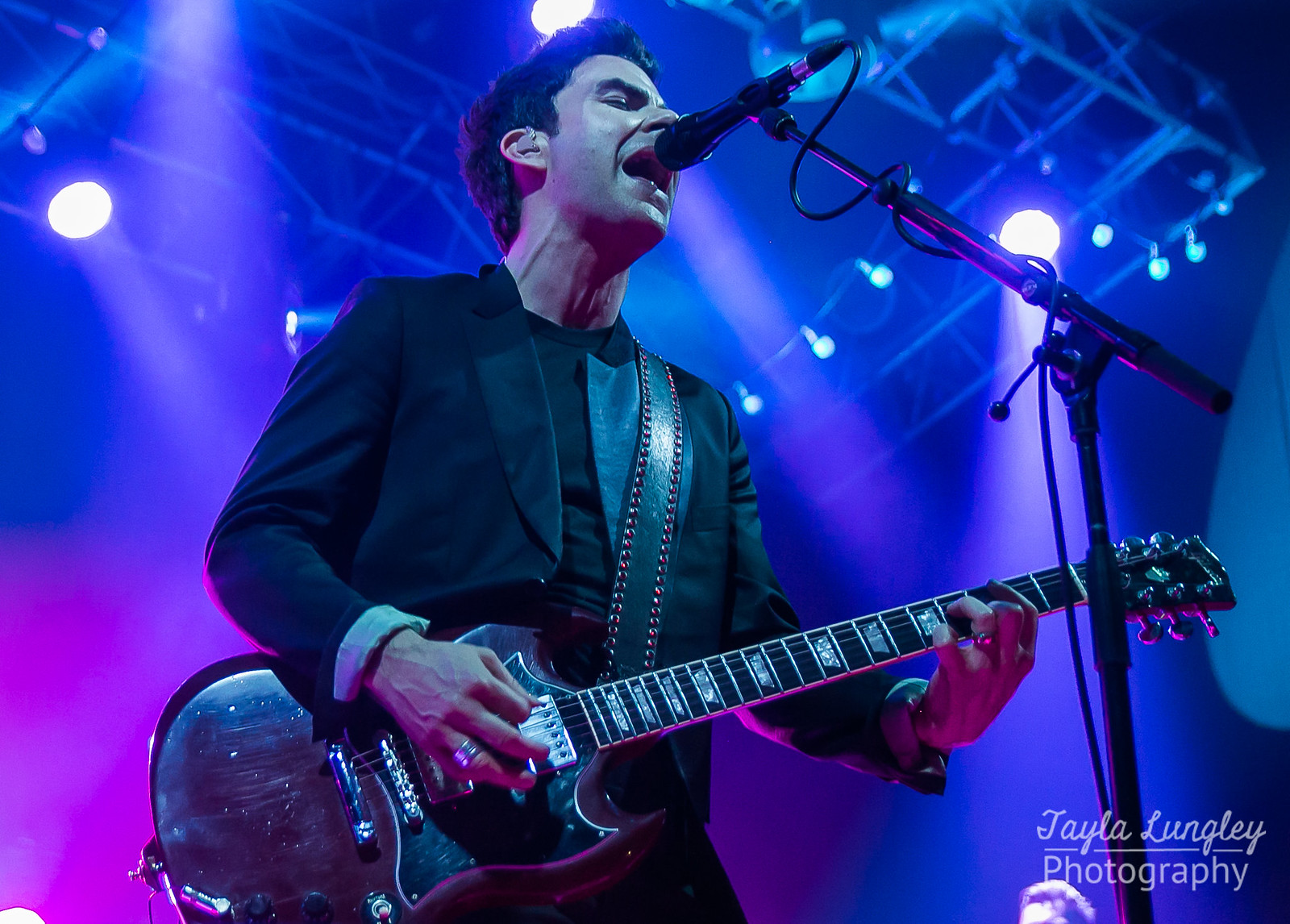This detailed image showcases a professional male singer performing on a very large stage, actively engaging with his audience in an action shot. The singer, appearing to be in his 30s or mid-40s, has short black hair and is in good shape. He is dressed entirely in black, wearing a black blazer, a black t-shirt, black pants, and a black leather strap adorned with sequins. His right sleeve is slightly rolled up, revealing a ring on his left hand, which is positioned on the neck of his black, possibly dark cherry rosewood Gibson SG electric guitar. The guitar features a black pickguard, silver pickups, and silver inlays on the fretboard. A sophisticated microphone setup extends from the bottom right corner of the image, arching towards his mouth, which is open as he sings into it. The background of the stage is bathed in a mix of bluish and purplish lights, with spotlights beaming down and creating a vibrant atmosphere. Over his right shoulder, a prominent spotlight shines, and the upper portion of the image hints at the support structure for the lighting rig. In the bottom right corner, a watermark credits "Taylor Lungley Photography," adding an artistic touch to the image.